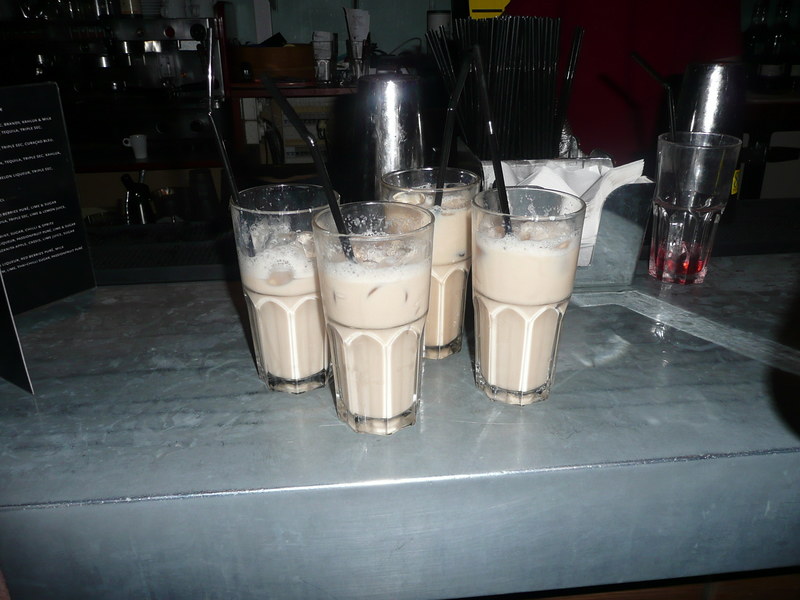In the image, four large, milky beige drinks adorned with black straws rest on a shiny metal bar countertop. Each glass is filled almost to the top, with a layer of foam capping the thick, icy liquid within. The scene is set in a bar or diner environment, with a box of napkins and a bundle of straws visible on the left, along with a menu and an empty glass containing a hint of red liquid, possibly cranberry juice. In the background, bar shakers and bottles, which might include liquor, contribute to the ambiance. The drinks appear ready to be served, encapsulating a bustling yet organized bar setting.